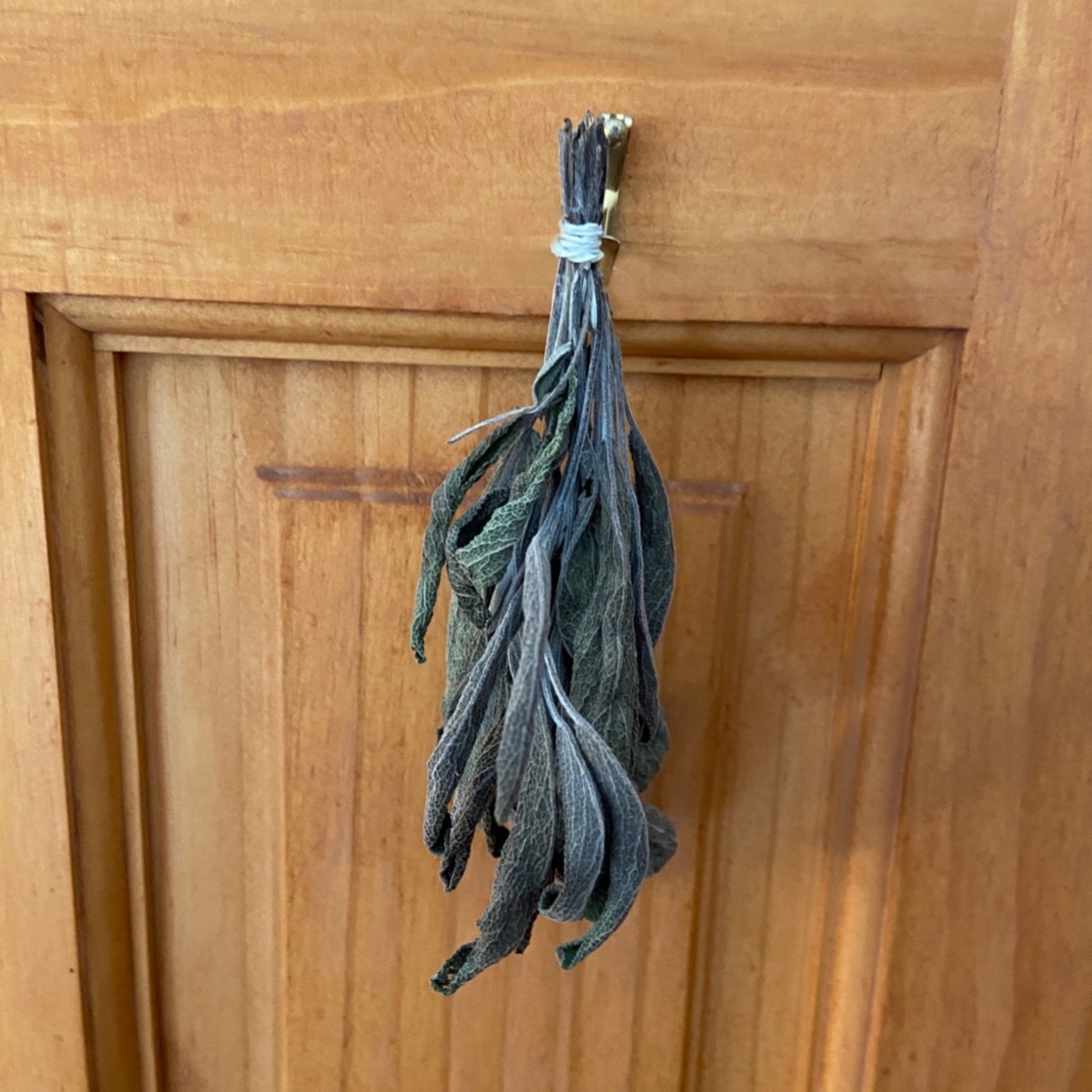In the image, a rustic wooden cabinet door, its light brown and tan hues muted by the central inset panel, serves as the backdrop for a bundle of dried foliage. The foliage, tied together at their stems with a light blue rubber band, hangs upside down, cascading down the door. The leaves, in shades of gray, purple, and bluish-green, exhibit signs of wilting, their ends curled and crisp from dryness. The bundle, resembling the form of a feather duster, occupies the middle of the door, drawing the eye to its delicate interconnected stems. There's also a hint of metal behind the dried leaves, adding a subtle industrial touch to the otherwise earthy scene. No text or explanation accompanies the image, leaving the purpose and story behind the arrangement to the viewer's imagination.